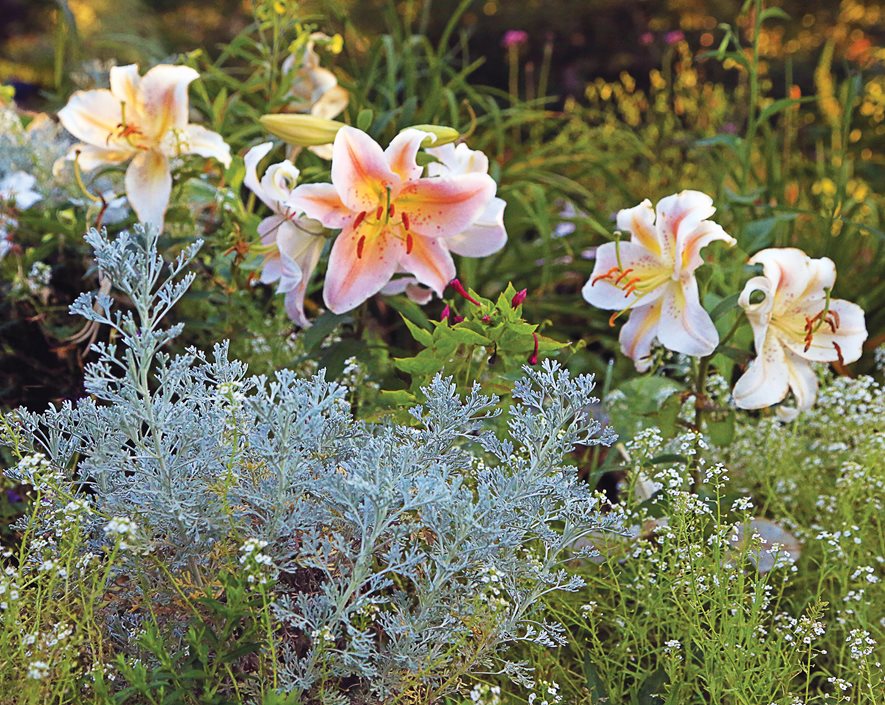The image captures a vibrant garden scene with a variety of flowers and plants. Central to the picture are striking white flowers with pink veins in their petals. These flowers have yellow and red inner petals surrounded by tubular red stamen-like structures, giving them an exotic appearance. The white blossoms, resembling lilies, transition from a darker pink toward the center to white at the tips. Below these central flowers are bluish-green ferns and small, delicate white flowers that resemble baby's breath, often used as fillers in bouquets. In the lower part of the image, more white flowers with tiny tips can be seen. The background is a blur of colors, with distorted greens, yellows, oranges, and purples, hinting at tropical plants and other flowers. The upper right corner of the image is darker, with purples becoming more pronounced. This garden scene is lush and teeming with life, showcasing a rich tapestry of floral beauty.